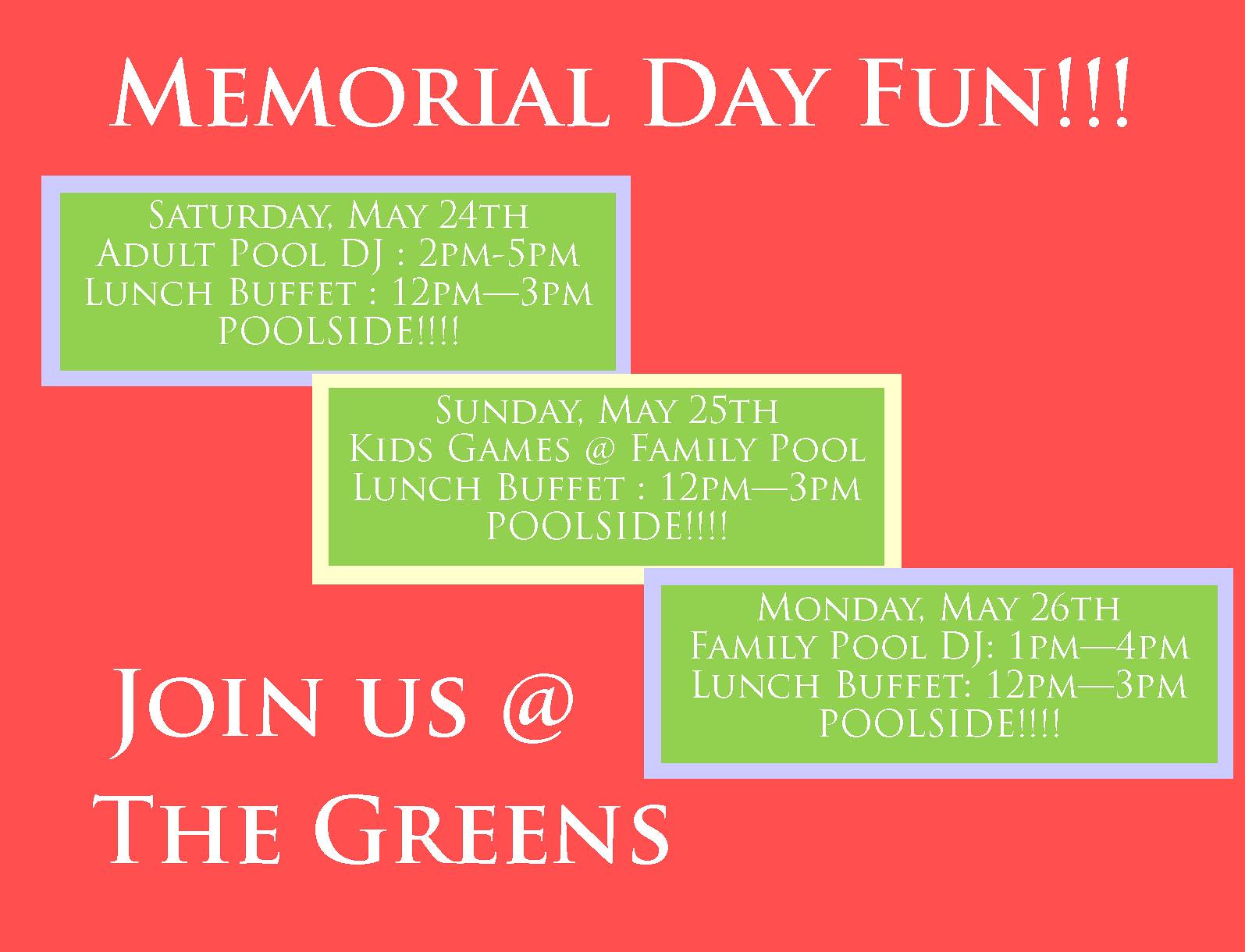The image features a vibrant, bright red background with a prominent Memorial Day event announcement. At the top, in large white font, it exclaims, "Memorial Day Fun!!!". Below, there are three green rectangles lined up vertically that detail the three-day celebration at The Greens. 

- The first rectangle announces activities for "Saturday, May 24th", including an "Adult Pool DJ" from 2PM to 5PM, and a "Lunch Buffet" available from 12PM to 3PM, all happening poolside.
- The second rectangle details "Sunday, May 25th", featuring "Kids Games at Family Pool" and a "Lunch Buffet" from 12PM to 3PM, also poolside.
- The third rectangle highlights "Monday, May 26th" with a "Family Pool DJ" from 1PM to 4PM, and again a "Lunch Buffet" from 12PM to 3PM, poolside.

At the bottom left corner, in white text, the invitation reads, "Join Us at the Greens." This festive graphic design image emphasizes a fun-filled, three-day Memorial Day celebration with various activities and meal times clearly noted.